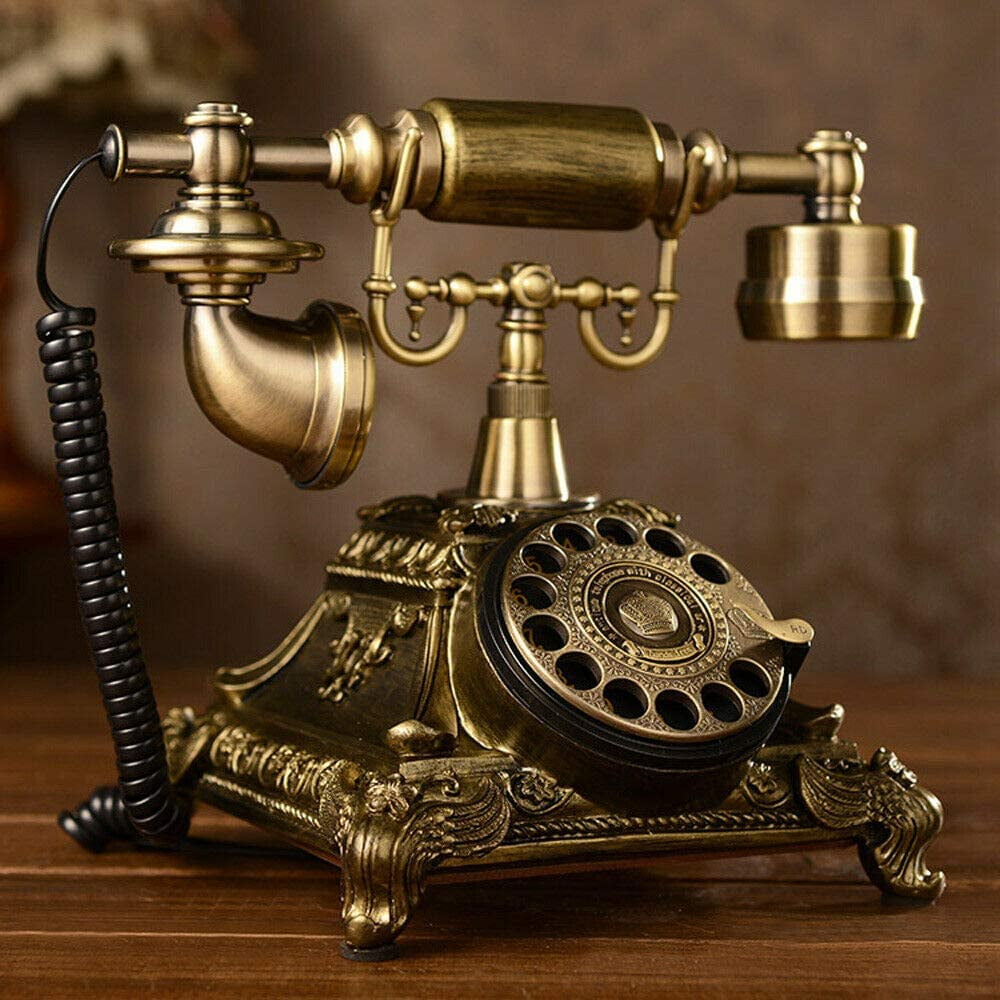In this indoor photographic setting, an antique-style rotary phone takes center stage. This phone, designed to mimic a 19th-century artifact, is crafted entirely out of metal with a lustrous bronze or brass finish. It stands on an intricately designed square base, supported by four dainty feet. The base features a rotary dial with small, unreadable print at its center, surrounded by numbers meant to be dialed with one's finger. A pole rises from the base to cradle the phone's receiver, which consists of a curved, cylindrical earpiece and a matching curved mouthpiece. The receiver is connected to the base by a coiled black cord.

The entire setup rests on a varnished, dark brown hardwood desk, which contrasts slightly with the medium brown, out-of-focus background. Off to the upper left corner of the image, a lighter brown, possibly a lamp shade, adds a touch of variance to the otherwise monochromatic blur. The overall aesthetic suggests a blend of antique elegance and modern reproduction, giving the phone an almost timeless appearance despite its old-fashioned design.